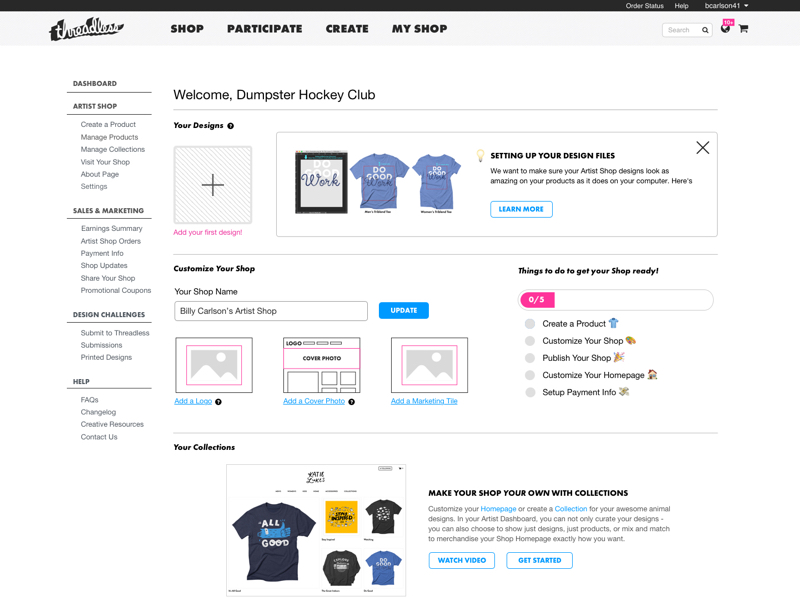Screenshot of a web page with a black header at the top displaying "Order Status Help" alongside a username. Below the header, navigation options include "Threadless," "Shop," "Participate," "Create," and "My Shop." On the left side, a vertical menu lists several sections: "Dashboard," "Artist Shop," and subcategories such as "Create a Product," "Manage Product," "Manage Collection," "Visit Your Shop," "About Page," "Setting," "Sales and Marketing," "Earnings Summary," "Artist Shop Orders," "Payment Info," "Shop Updates," "Share Your Shop," "Promotional Coupons," "Design Challenges," "Submit Threadless Submission," "Printed Design," "Help FAQs," "Creative Resources," and "Contact Us." On the main panel to the right, a welcome message "Welcome, Dumpster Hockey Club" is displayed with two T-shirt images underneath, and a section titled "Setting Up Your Design Files."